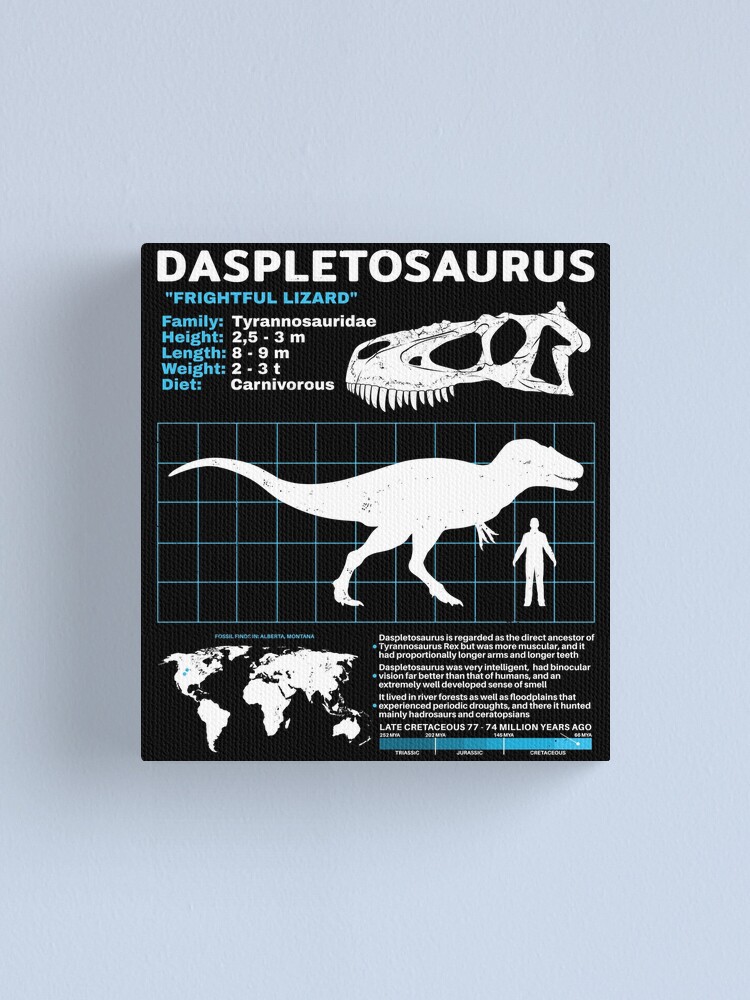Displayed against a light gray wall is an informative black poster about the Daspletosaurus, also known as the "frightful lizard." The top of the poster features "Daspletosaurus" in bold white letters and "frightful lizard" in blue quotes. The poster provides detailed information about the dinosaur's classification, including its family, Tyrannosauridae, and specifics such as height (2.5-3 meters), length (8-9 meters), weight (2-3 tons), and diet (carnivorous), with each metric highlighted in alternating blue and white text.

Central to the poster is a white silhouette of the Daspletosaurus juxtaposed with a human silhouette for size comparison, both set against a light blue grid that comprises approximately five horizontal by eleven vertical lines. Detailed illustrations of the dinosaur's skull and teeth are positioned to the right of the textual information.

Below this central imagery is a concise world map highlighting the geographical distribution of the Daspletosaurus, also rendered in white against the black background. The poster also includes paragraphs of descriptive text and a blue line graph with white markers, though these sections are not fully legible. This educational and visually engaging display is akin to exhibits found in museums or scholarly publications.